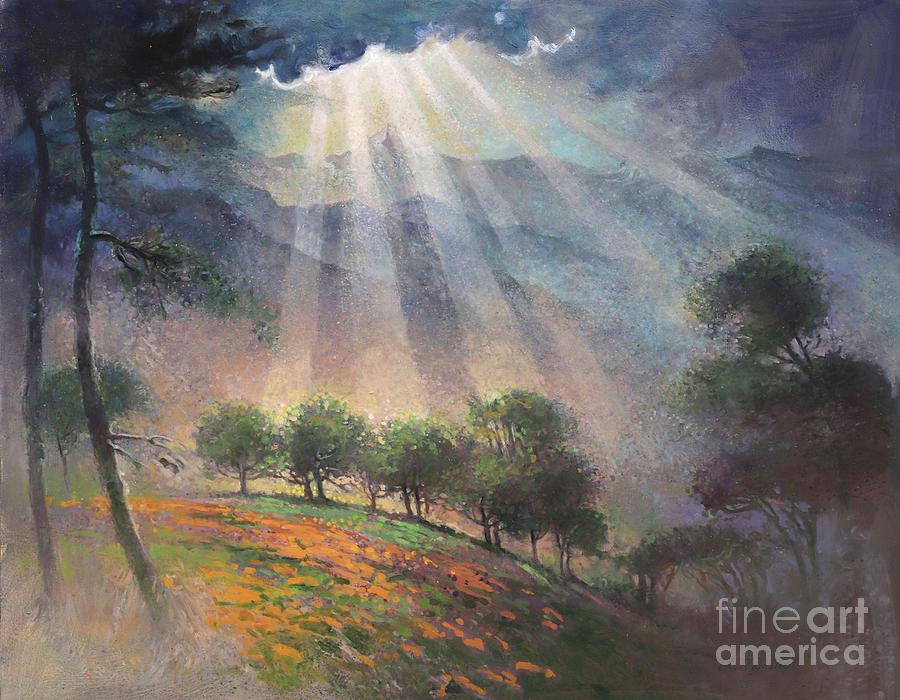This painting, showcased by Fine Art America, depicts a serene, semi-realistic landscape that evokes the stylistic elements of impressionism. It captures a sparsely wooded area with scattered trees of varying sizes, some in the foreground and some in the background. The green grass is intermittently highlighted with shades of orange, suggesting either flowers or the play of light on the landscape. 

Above, the sky is primarily a gray-blue, with a break in the clouds revealing hues of lighter blue, green, and yellow. Six distinct sunbeams penetrate through this opening, casting a mesmerizing light onto the trees and the grassy hill below. The sunbeams are accentuated by white rim lighting around the clouds, creating a radiant effect as they beam downwards. Subtle details, such as patches of dirt on the hill and the vibrant colors in the grass, add depth and texture to the scene. 

The painting's print is situated in the bottom right corner, and the remarkable rendering of this outdoor setting showcases the artist's talent for capturing the interplay of light and nature's beauty.